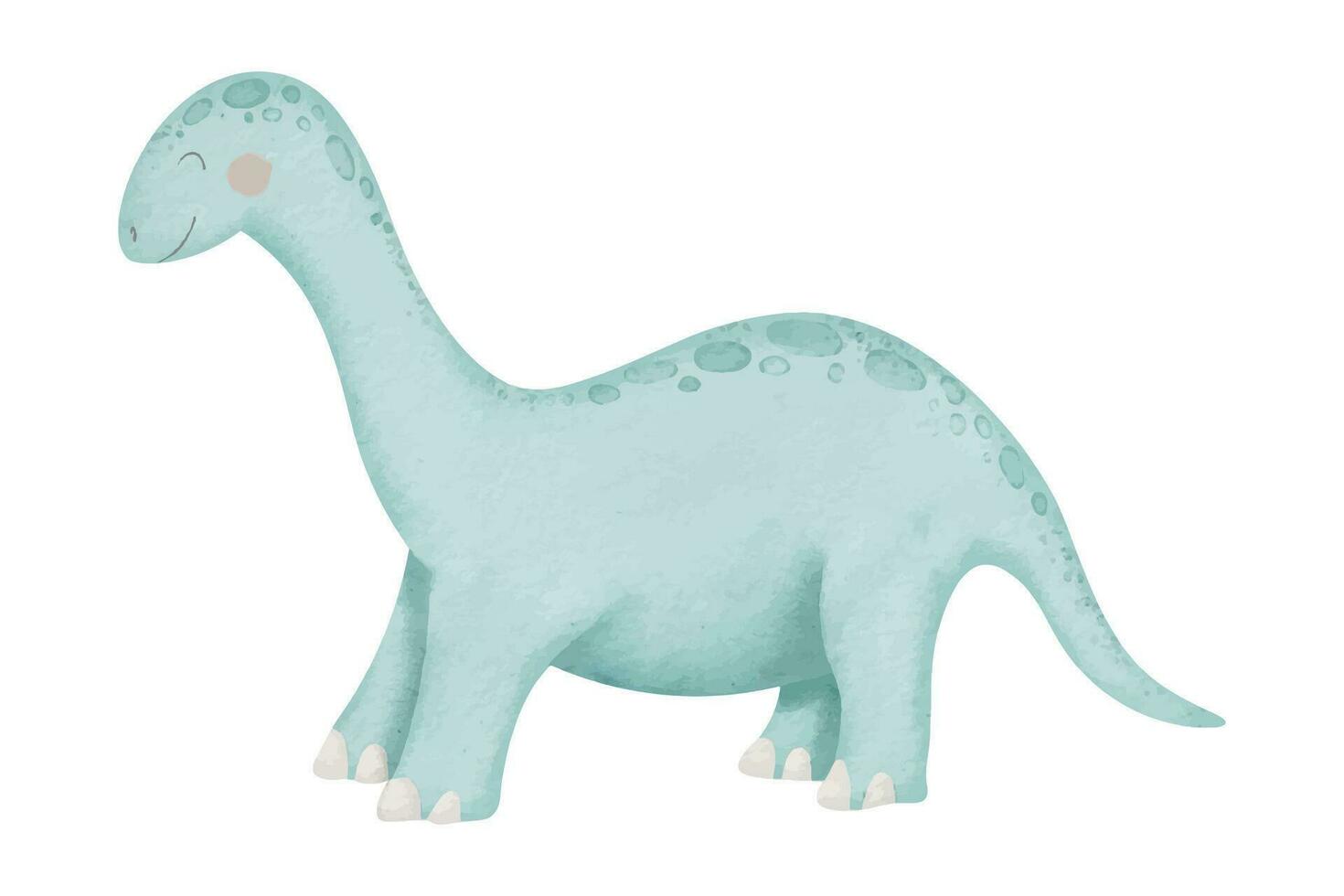This charming illustration features a whimsical, blue dinosaur reminiscent of those seen in children's books. The dinosaur, likely a Brachiosaurus with its large body, long neck, and small head, appears playful and inviting rather than frightening. It boasts a series of darker turquoise polka dots that run from the top of its head, down its neck, along its back, and to the tip of its thin, pointy tail. Its little feet have white hoof-like toenails, adding to its endearing appearance. The dinosaur is depicted with a joyful smile, eyes closed, and a single, outlined nostril, while its cheeks are adorned with rosy blush, enhancing its playful and friendly demeanor. The head is angled to the left and the tail to the right, capturing a moment of delightful stillness.